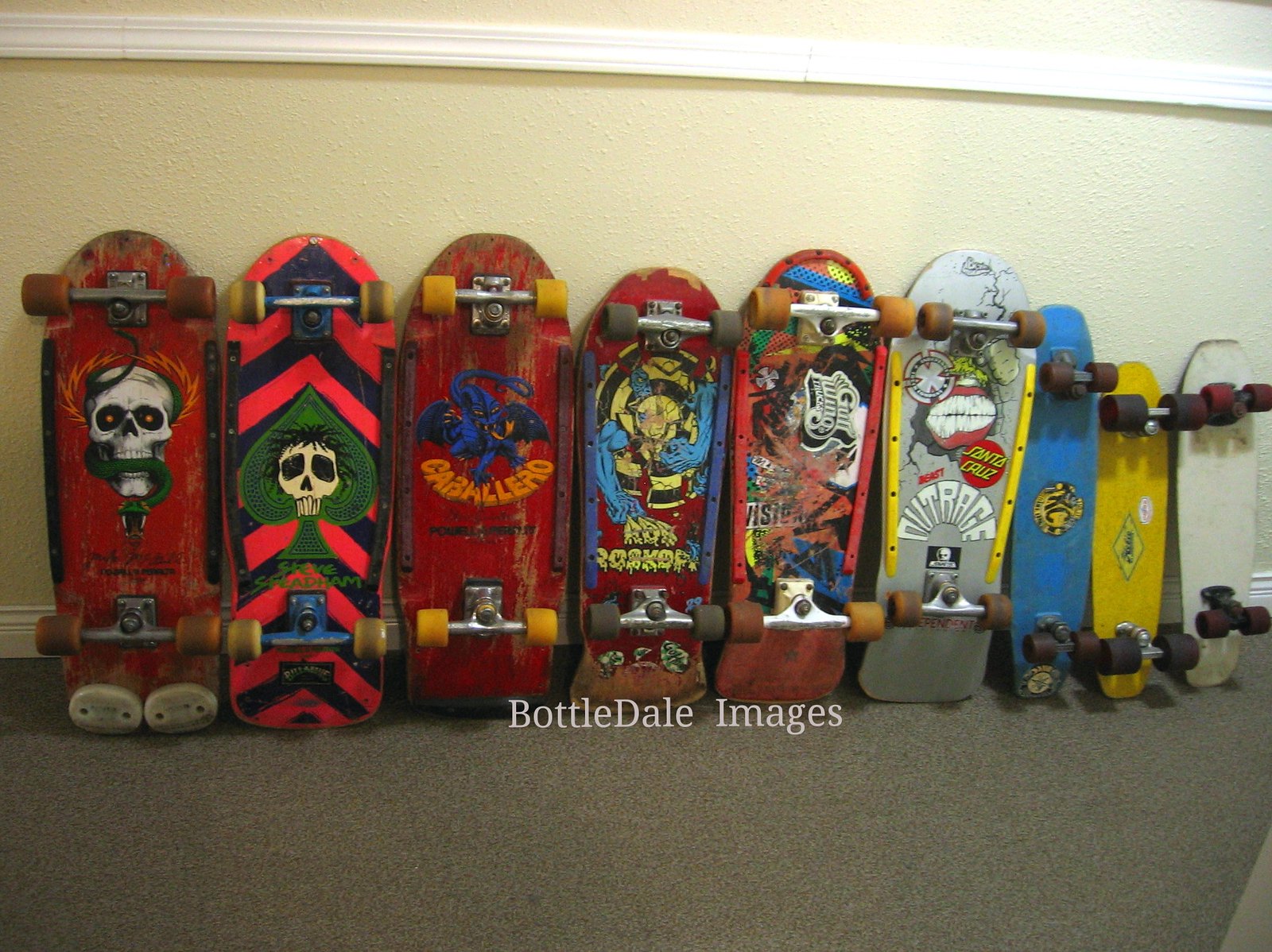In this detailed, indoor photograph, nine skateboards are lined up vertically against a cream-colored wall with white trim. The skateboards are positioned with their wheels facing the camera, resting on a brown-gray carpet. The image is in landscape orientation and captures the vibrant graphics on the underside of each skateboard. From left to right, the designs and colors vary: the leftmost features a white skull entwined with a black snake on a red background, followed by a green spade adorned with a white skull and orange-black stripes. Next is a blue creature labeled "Chalero," and then a blue illustration with an illegible figure and text. As we move further right, there is a skateboard with a zombie emerging from a target, a colorful abstract design, and one depicting a dog smashing through a wall with a grinning mouth and the word "Outrage." The smaller, classic-looking skateboards are positioned on the far right. White text near the bottom of the image reads "BOTTLEDALE IMAGES." Overall, each skateboard showcases unique logos and designs, contributing to a colorful and detailed composition reflective of modern and classic skate culture.